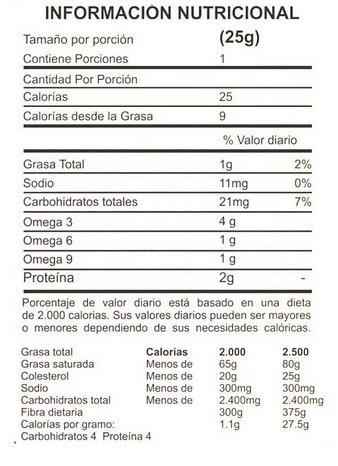This image displays a nutritional label written in Spanish, presenting a structured and comprehensive overview of the product’s nutritional components. The label is set against a white background with black text, ensuring clear readability. The title at the top of the label reads "Información Nutricional," which translates to "Nutritional Information." Below the title, the label details various nutritional elements, including calories, sodium, and carbohydrates. In addition to these, specific vitamins and minerals such as Omega-3, Omega-6, and Omega-9 fatty acids are mentioned. There is also a segment that indicates the protein content in the product. The label is systematically organized with horizontal black lines dividing different sections, making it easy to distinguish between various pieces of nutritional information.